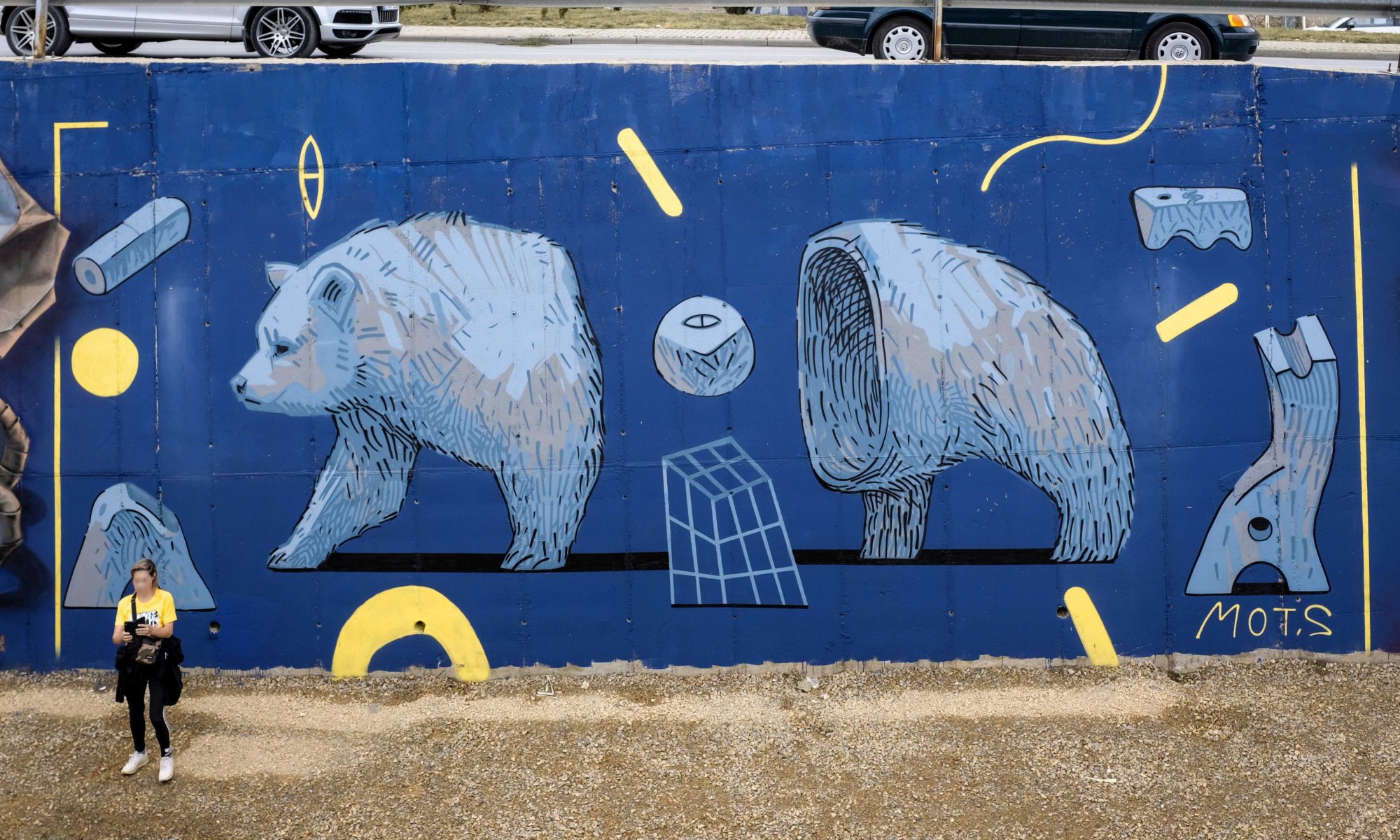The mural depicted in this image showcases a mesmerizing piece of art painted on the expansive side of a structure, likely a bridge rather than a building. The mural features a royal blue background, which expertly draws attention to the central figure of a grizzly bear. The bear, rendered in shades of light white and gray, is intriguingly presented with its body split in half. The left side of the bear reveals its head, presented in profile, while the right side displays the bear's posterior. This striking composition highlights the muralist's exceptional skill and mastery of the medium, transforming the structure into an enthralling canvas of wildlife artistry.